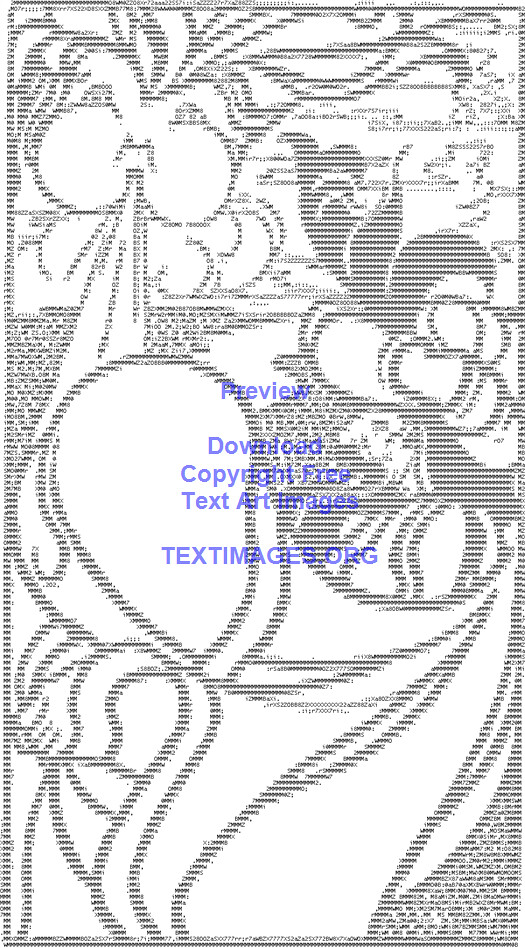This detailed black and white ASCII art illustration, set on a white background, is created entirely from black text characters, utilizing different shades and lines to form intricate visual elements. Dominating the scene is a whimsical depiction of a cloud with big cheeks and wavy hair, blowing a strong stream of wind from the upper left corner. Complementing this main feature, there's an array of other details: prominently, a large flower possibly resembling an orchid in the upper left, and another big flower in the bottom, with additional floral or botanical elements and wavy designs, potentially signifying water, scattered throughout. The illustration also includes a Sultan-like face in the bottom right corner, adding an exotic flair to the composition. Overlaying this art in the center is a succession of blue text that reads: "Preview," then a gap, followed by "Download," "Copyright-Free," "Text Art Images," and finally, "textimages.org."